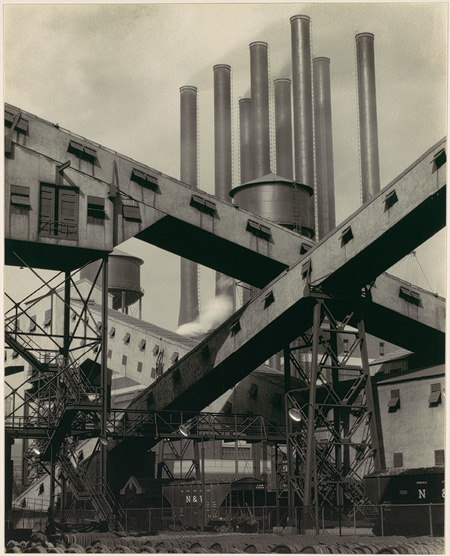The black and white photograph depicts a sprawling industrial facility, dominated by a complex arrangement of structures and machinery. In the foreground, rows of barrels lie in front of a chain-link fence, beyond which stand two large railway train cars designed for coal transport. These cars are flanked by an intricate scaffolding system, complete with a network of crisscrossing beams and multi-flight staircases that climb towards the sky. The central focus of the image is an expansive industrial building, replete with numerous windows and elevated walkways that resemble jet bridges on stilts. This building stretches across the middle of the frame, its metallic supports and hallways forming a labyrinthine pattern against the cloudy sky. Towering in the background, a series of smokestacks rise alongside several water towers, belching smoke that underscores the industrial nature of the scene. The entire setting is outdoors under a heavily clouded sky, encapsulating the stark, utilitarian atmosphere of this industrial plant.